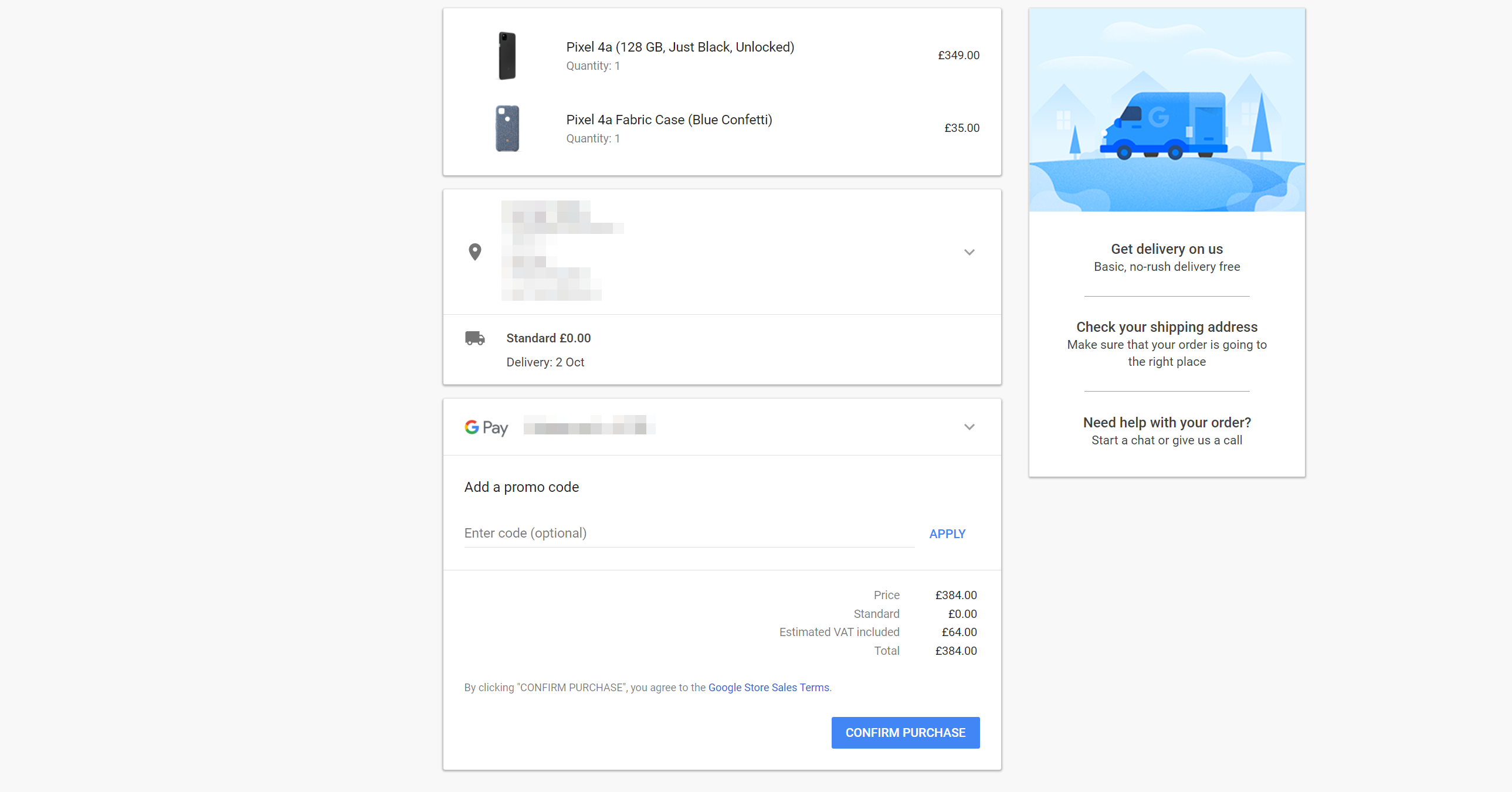The image depicts an online shopping cart interface for purchasing a Google Pixel 4a and related accessories. At the top, there is a listing for a Google Pixel 4a, which features 128 gigabytes of storage, is colored in "Just Black," and is unlocked, priced at £349. Accompanying this listing is a picture of the black smartphone.

Below the phone listing, there is an entry for the ‘Pixel 4a Fabric Case’ in the ‘Blue Confetti’ color, priced at £35, with an image of the blue fabric case next to it.

Further down, the section highlights that a pin icon is used to denote the shipping location, with personal information intentionally pixelated to ensure privacy. The shipping method is standard and free, signified by a delivery truck icon. The expected delivery date is October 2nd.

The checkout section includes the Google logo followed by a Google Pay option, where credit card details would typically be displayed but are pixelated for privacy. Below, there is an option to enter a promo code. The price breakdown shows the item subtotal of £349, with shipping being free, an estimated VAT of £64, totaling £384.

At the bottom, a statement mentions that by clicking the "Confirm Purchase" button, the buyer agrees to the Google Store sales terms, and there is a blue "Confirm Purchase" button below this statement.

On the right-hand side, a blue van icon with the letter 'G' for Google indicates a message about "Get Delivery On Us" with basic, no-rush delivery being free. It advises customers to check their shipping address to ensure the order is going to the correct location and provides options for customer support through a chat or a phone call if help is needed with the order.